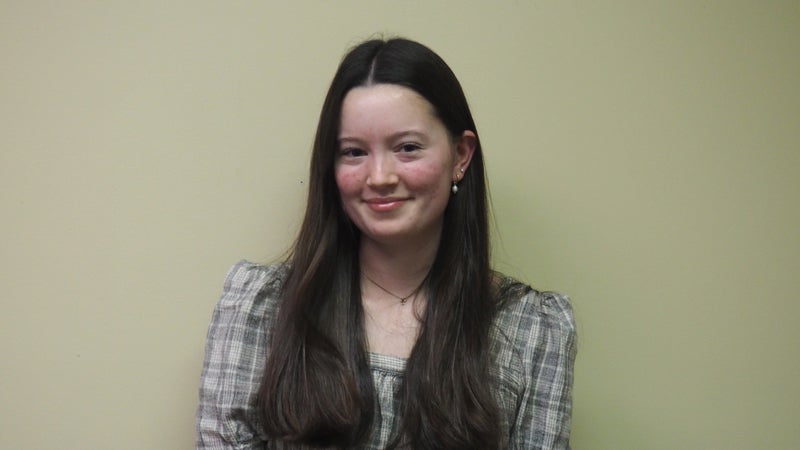This horizontal color photograph features a young Caucasian woman standing in front of a taupe-colored wall. Seen from above the elbows up, she has a slight, pleasant grin on her face with red cheeks. Her dark brown hair, parted in the middle, flows down to her breasts, with one side tucked behind her ear, revealing at least two earrings, including a pearl earring. She wears a plain gray dress with a square neckline adorned with white vertical and horizontal lines, resembling a checkered pattern. Around her neck is a delicate, thin black necklace. Her overall expression is happy and warm, contributing to the inviting nature of the photograph.